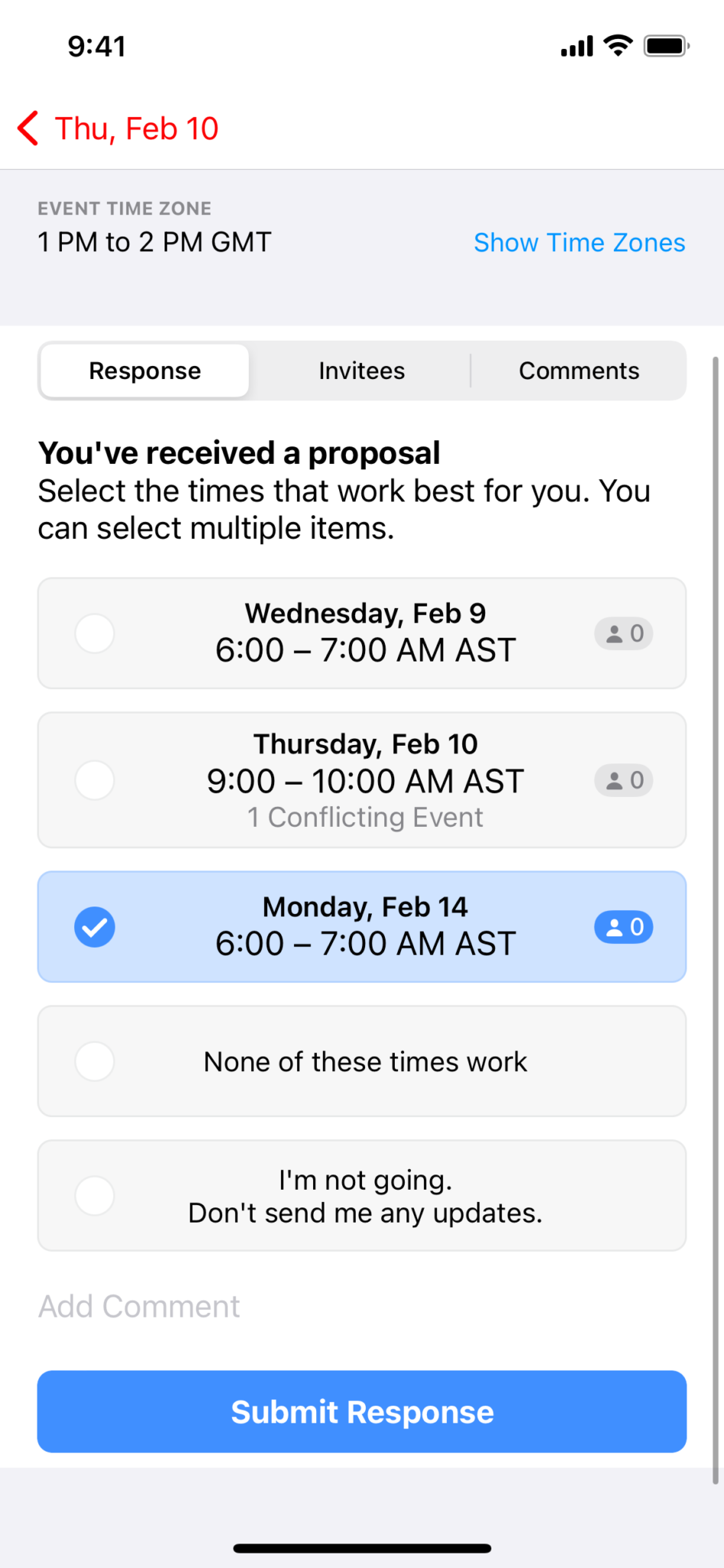This smartphone screenshot displays the interface for responding to an event proposal. At the very top, there is a section showing an event scheduled for "Thursday, February 10," with a red date and a back arrow on the left. Beneath this, a gray bar labeled "event time zone" appears on the left, while the event time "1pm to 2pm GMT" is noted below. On the right side of the gray bar, "show time zones" is prominently displayed in blue text.

Below the time zone information, there are three side-by-side buttons labeled "Responses," "Comments," and another option not specified but likely similar, with "Responses" being highlighted in white while the others are grayed out.

Further down, there is a message informing the user that they have received a proposal and instructing them to "select the times that work best for you; you can select multiple items." A list of available dates follows, including:

- Wednesday, Feb 9
- Thursday, Feb 10
- Monday, Feb 14

Each date is accompanied by a selectable checkbox; the date "Monday, Feb 14" is highlighted in blue with a corresponding blue checkmark to its left. At the bottom of the list, there are additional options reading "None of these times work" and "I'm not going, don't send me any updates."